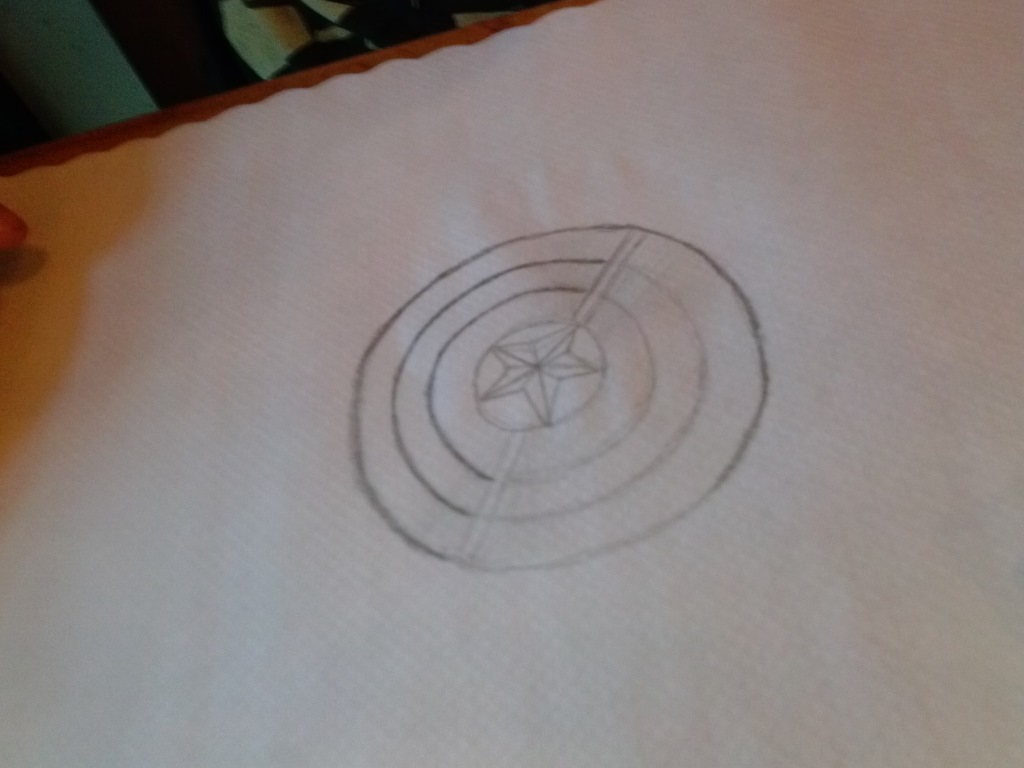The photograph captures a detailed pencil sketch on a white, wavy-edged medium, possibly a sheet of paper or fabric, placed on a wooden table. The background features a green wall adorned with plants, adding a touch of natural ambiance. The central artwork, reminiscent of Captain America's shield, consists of several concentric circles encircling a five-pointed star. A distinct line intersects the concentric circles, enhancing the geometric intricacy of the design.